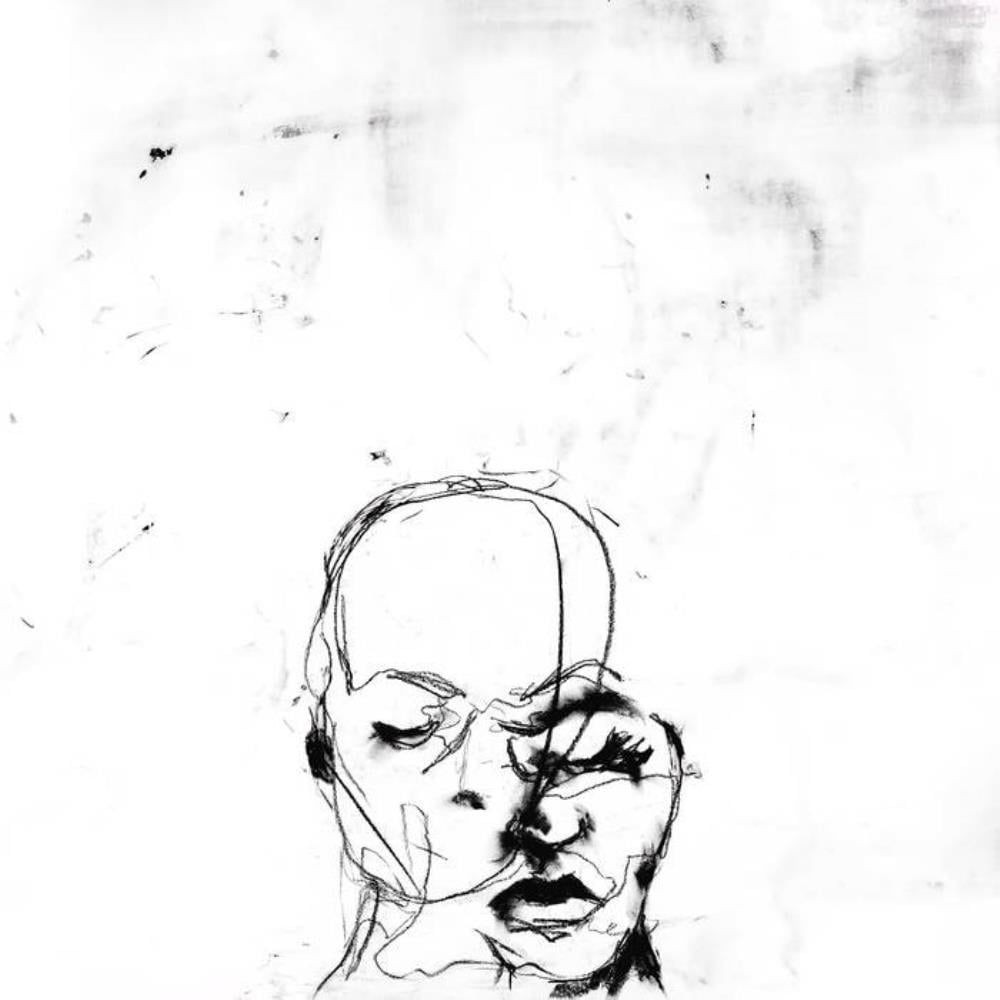This black and white modern abstract artwork is a detailed line drawing of two intertwined faces, blending seamlessly into one another. The primary face, identifiable as a woman's, is intricately detailed, showcasing features such as lips, eyes, nose, eyebrows, and a neck with noticeable shadowing. Overlapping this face is a second head, less detailed, serving as a silhouette with minimal features like eyes and a nose. The merging of these faces creates an evocative, surreal image. The background, primarily white, is accentuated with faint gray paint strokes and swirls, adding a subtle texture. Additionally, black dots and flecks of paint are scattered around the gray accents at the top, enriching the overall composition with a grunge-like texture that enhances the abstract nature of the piece.